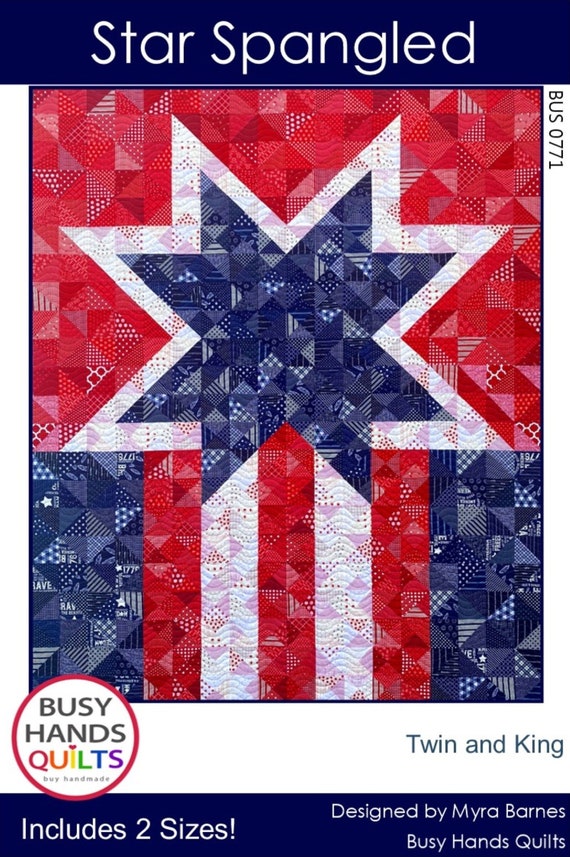This image appears to be an advertisement for a quilt named "Star Spangled" from Busy Hands Quilts, designed by Myra Barnes. At the top of the image, a dark blue banner displays the words "Star Spangled." The quilt itself features a patriotic red, white, and blue design. Central to its composition is a large blue star, bordered in white, set against a red background. Descending from the star are two white stripes, flanked by dark blue rectangles in the bottom left and right corners of the quilt. The quilt's intricate patchwork incorporates various shades and patterns within the red, white, and blue color scheme, with some patches showing hints of darker reds, and others featuring designs within the blue and white areas. Encapsulating the quilt’s label in a red-outlined circle at the bottom, the label reads "Busy Hands Quilts," with the word "Quilts" displayed in rainbow lettering. To the right of the circle, the text specifies that the quilt is available in twin and king sizes, and includes an identification number, BUS0771. This detailed and vivid design positions the quilt as both functional and decorative, suitable for enhancing any bedding collection.